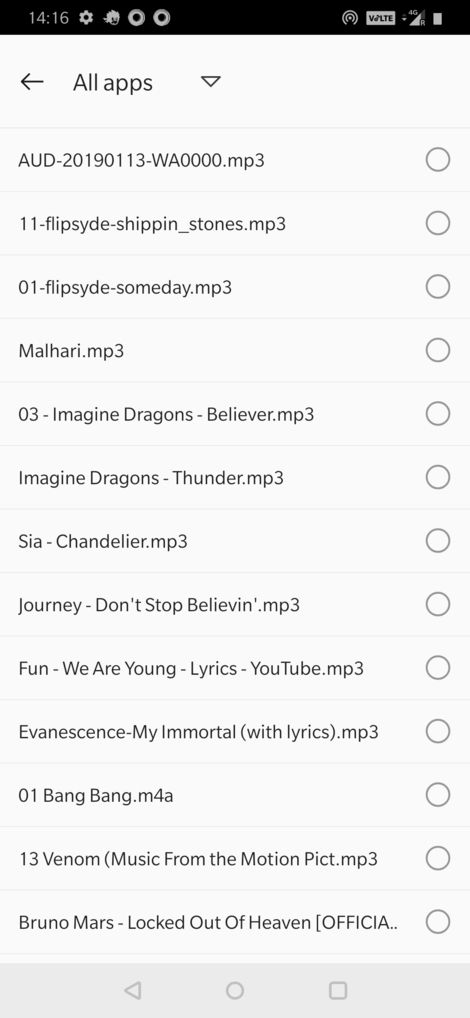The screenshot showcases a mobile phone display. At the top, there is a black status bar featuring white text. On the left side of this bar, the time is displayed as "14:16," and to the right, there is a settings icon. The upper right corner of the status bar shows a fully charged battery, 4G signal strength, and WLTE connectivity. 

Below the black status bar, there's a white background section. At the top of this section, "All apps" is visible, accompanied by a pull-down arrow to its right. Listed beneath this are three music files, each labeled with its format and artist information. From top to bottom, they are: "sia - chandelier.mp3," "journey - don't stop believing.mp3," and another file in the format "mp3."